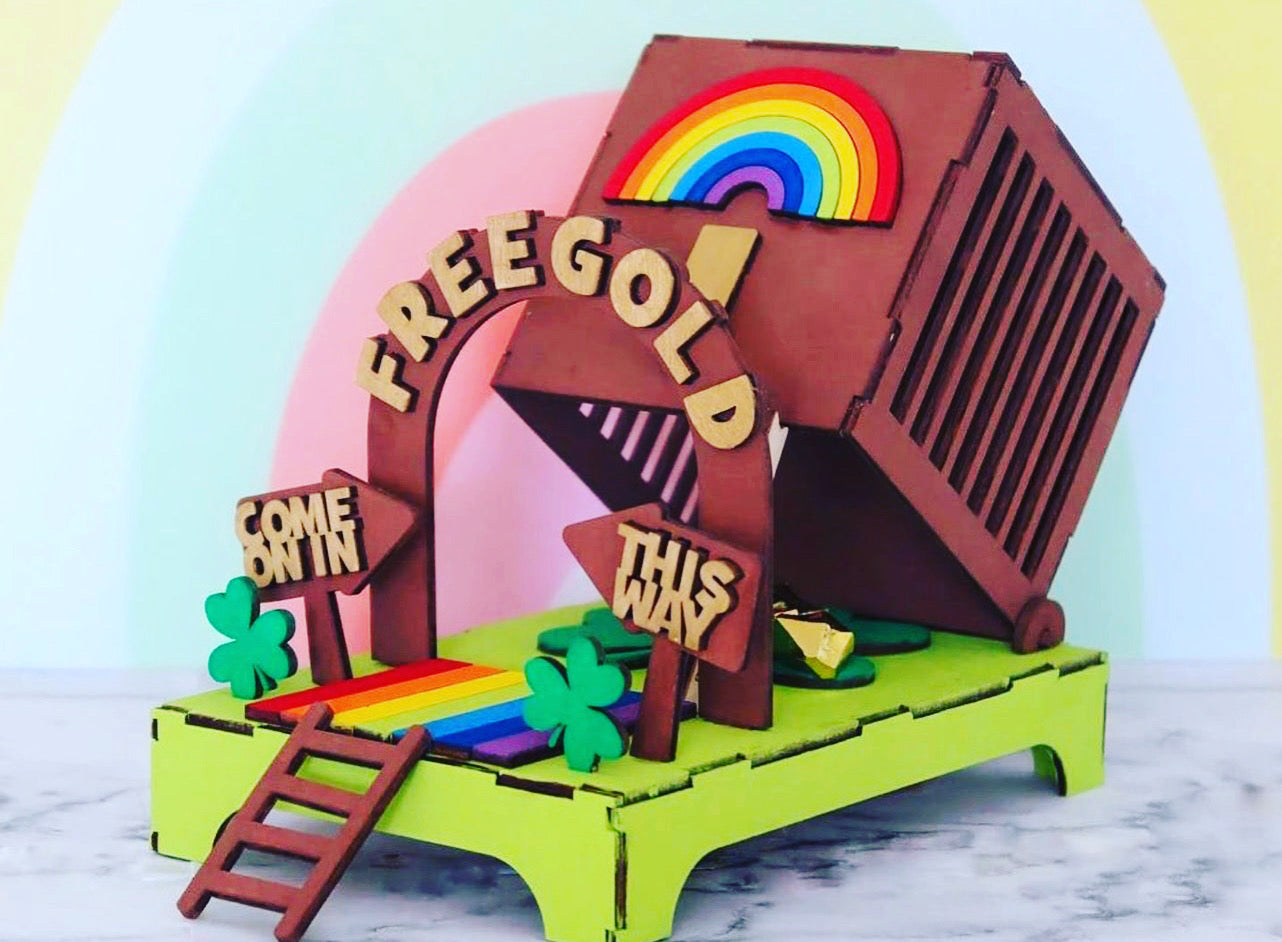This image showcases a whimsical, leprechaun trap set on a white marble surface with faint black lines, positioned in front of a rainbow-colored wall. At its base, a green cardboard platform mimics a stage. A small brown ladder on the front left leads up to a rainbow-colored welcome mat, flanked by two three-leaf clovers. On either side of the mat, signs with arrows point towards each other, reading "Come on in" on the left and "This way" on the right. Centered above the mat is a red or brown arch with the words "Free Gold" written in tan letters. Under this arch, partially obscured, sits what appears to be some gold, promising treasure but setting the scene for the actual trap. Hovering above, a brownish wooden box, adorned with a half-circle rainbow, stands ready to drop when the gold is disturbed, effectively capturing the unsuspecting leprechaun underneath. The entire setup is artistically rendered to evoke both playfulness and a sense of adventure.